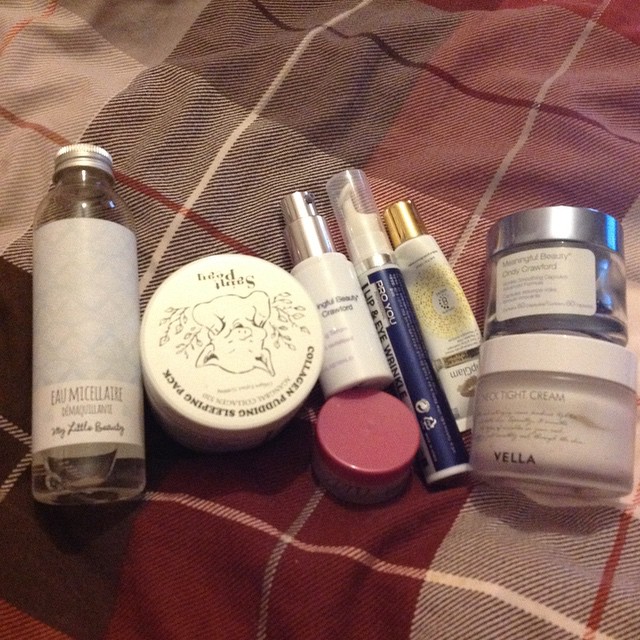In the image, the foreground is adorned with a cloth featuring a mix of red, gray, and light red hues. Centrally displayed on this cloth are various beauty products. At the heart of the arrangement are several lipsticks and creams, meticulously placed on a panel. Surrounding these items is an assortment of diverse containers: in the background, there's a glass bottle with a white label and a silver cap, alongside another bottle tinted in red. Additionally, a white bottle and a blue tube-like container can be seen. On the right side of the image, there are three cream containers - one in silver, another in white, and a third featuring a white tube with a gold cap. This intricate display of cosmetics is accentuated by the colorful cloth beneath them.